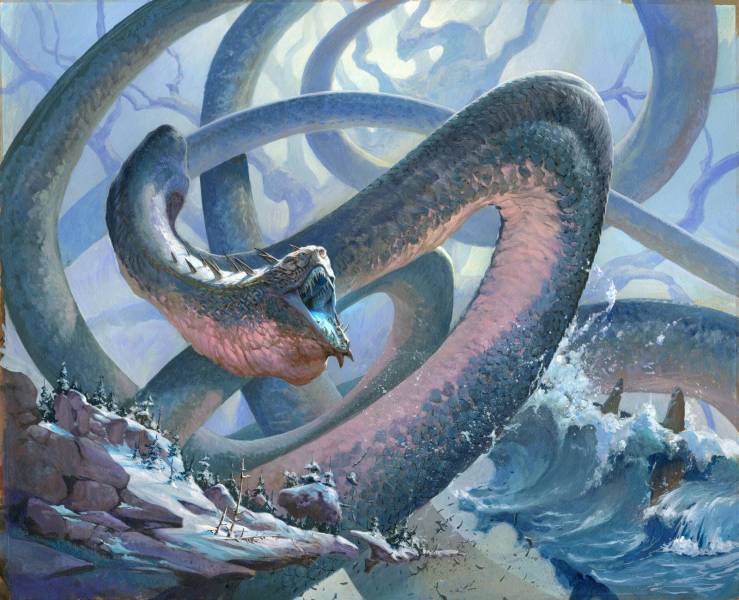The image depicts a breathtaking and otherworldly scene that evokes the essence of fantasy. Dominating the frame is an enormous, serpentine creature with menacing features. The beast displays an open mouth bristling with massive teeth, a tongue protruding, and a neck adorned with sharp spikes. Its immense, sinewy body extends and splashes into the churning ocean, creating dramatic waves and white foam. The water, tinted in hues of blue and silver, crashes against the jagged rocks to the left, where a group of small, dark blue-clad soldiers are positioned. These soldiers, appearing minuscule in comparison to the monstrous serpent, are outfitted with spears and preparing for a daunting battle. The backdrop is a misty, cloud-laden sky, enhancing the mystical ambiance. To the right, amidst the turbulent waters, lie capsized brown canoes, one of which still contains a stranded occupant. The mythical snake, with its grayish exterior and pink underbelly, looms hundreds of feet tall, creating a dire and tense atmosphere as it seemingly gears up for an imminent assault on the tiny figures below.